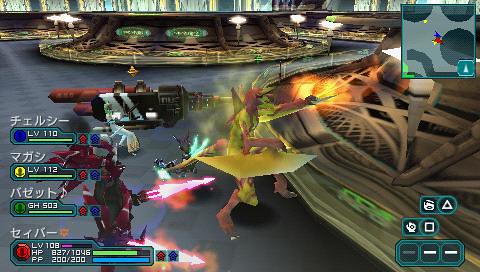The image is a detailed screenshot from an RPG-like combat video game with early 2000s to late 90s graphics, reminiscent of PlayStation 2 or 3 era but not necessarily from a PlayStation game. The display primarily features four distinct monster characters, each indicated by Japanese Katakana names and various levels, such as one being level 110, another level 112, and another labeled GH503. 

At the center, the protagonist is a peculiar yellow creature with red hair, forearms, and legs, equipped with blades on each arm, currently seen attacking what appears to be a structure exhibiting intricate weaving patterns. To the left, another character is clad in a red robotic suit with spikes and wielding two glowing pink daggers. In the background, another figure, possibly wearing a white suit, is seen holding a large black and white object, maybe a cannon or drill. 

The heads-up display (HUD) provides significant information: in the bottom left, one character's stats are shown, displaying level 108, HP 827/1046, and PP 200/200. The top-left corner features a mini-map with circular engravings marking character positions. The bottom right corner shows button mappings such as triangle and square for different actions and what seems like three inventory slots. The left of the screen lists four players by color-coded icons with blue, yellow, green, and red, including red and blue buffs next to their names. The game environment includes green pillar-like structures and multiple windows with intersecting lines, contributing to an intricate, immersive atmosphere.